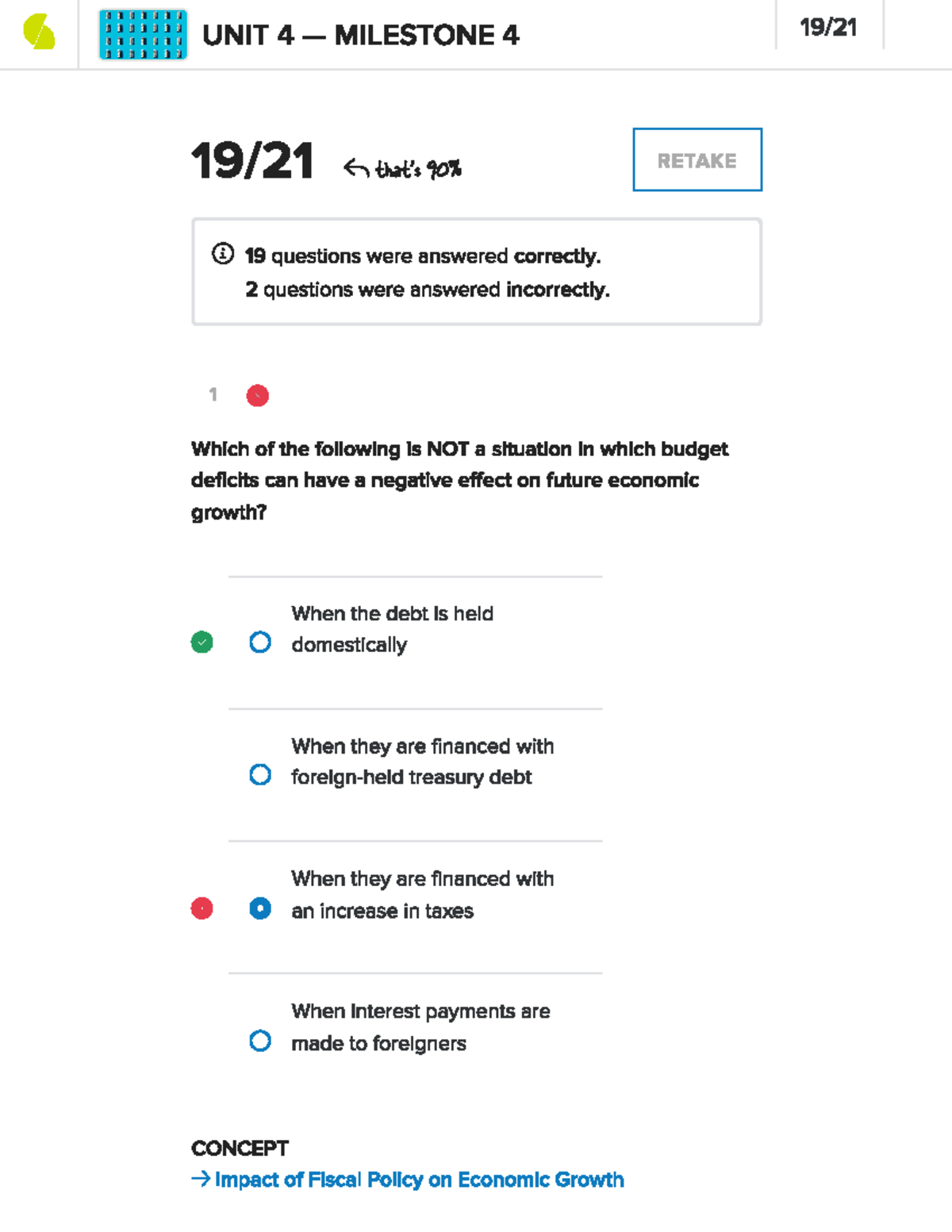Here's a cleaned and detailed caption for the image:

---

This image appears to be a screenshot from an educational website or app, likely depicting the results of an online exam. In the upper left-hand corner, a curved, light green logo is visible, alongside a rectangle composed of interlocking light blue and dark blue squares, giving it a woven appearance. In white text, the image displays "Unit 4, Milestone 4," followed by "19/21." Below this, a thin grey line separates the header from the main content.

Centrally located is a score display, "19/21," which translates to 90%, with a "retake" option to the right that is greyed out and outlined by a blue rim. This suggests that the option to retake the exam is currently not available. Underneath, a detailed summary indicates "19 questions answered correctly" and "2 questions answered incorrectly," contained within a grey rectangle.

The image also includes a sample question: "Which of the following is not a situation in which budget deficits can have a negative effect on future economic growth?" Four options are listed:

1. When the debt is held domestically (not ticked, likely the correct answer)
2. When they are financed with foreign-held treasury debt (not ticked)
3. When they are financed with an increase in taxes (ticked but incorrect)
4. When interest payments are made to foreigners (not ticked)

Below the question, a concept is referenced, with a blue arrow pointing to it labeled "Impact of fiscal policy on economic growth."

---

This caption aims to provide a detailed and clear description of the contents and context of the screenshot.